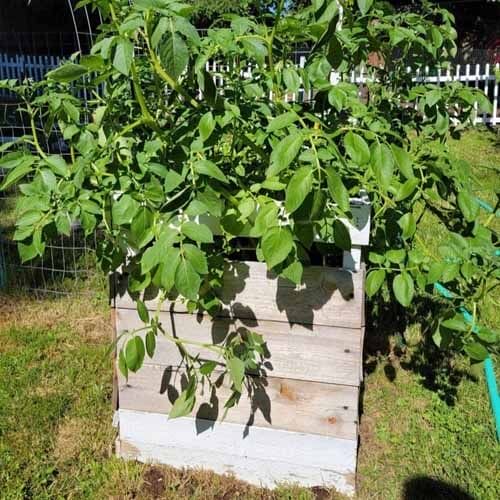This photograph captures a backyard garden scene with a wooden planter box prominently placed in the center. The rectangular planter, constructed from approximately five nailed wooden slats, each about a foot and a half long, contains a lush, green plant with leaves resembling those of a tomato plant, though its exact species is uncertain. The foreground features a mix of green and brown grass, while the background displays a white picket fence running the width of the image. Just behind the planter, a chicken wire fence is visible, further emphasizing the garden's layout. To the right, a green garden hose lies on the ground, hinting at regular gardening activity. The photograph suggests an avid gardener's devotion to their backyard oasis, with additional trees adding to the verdant backdrop.